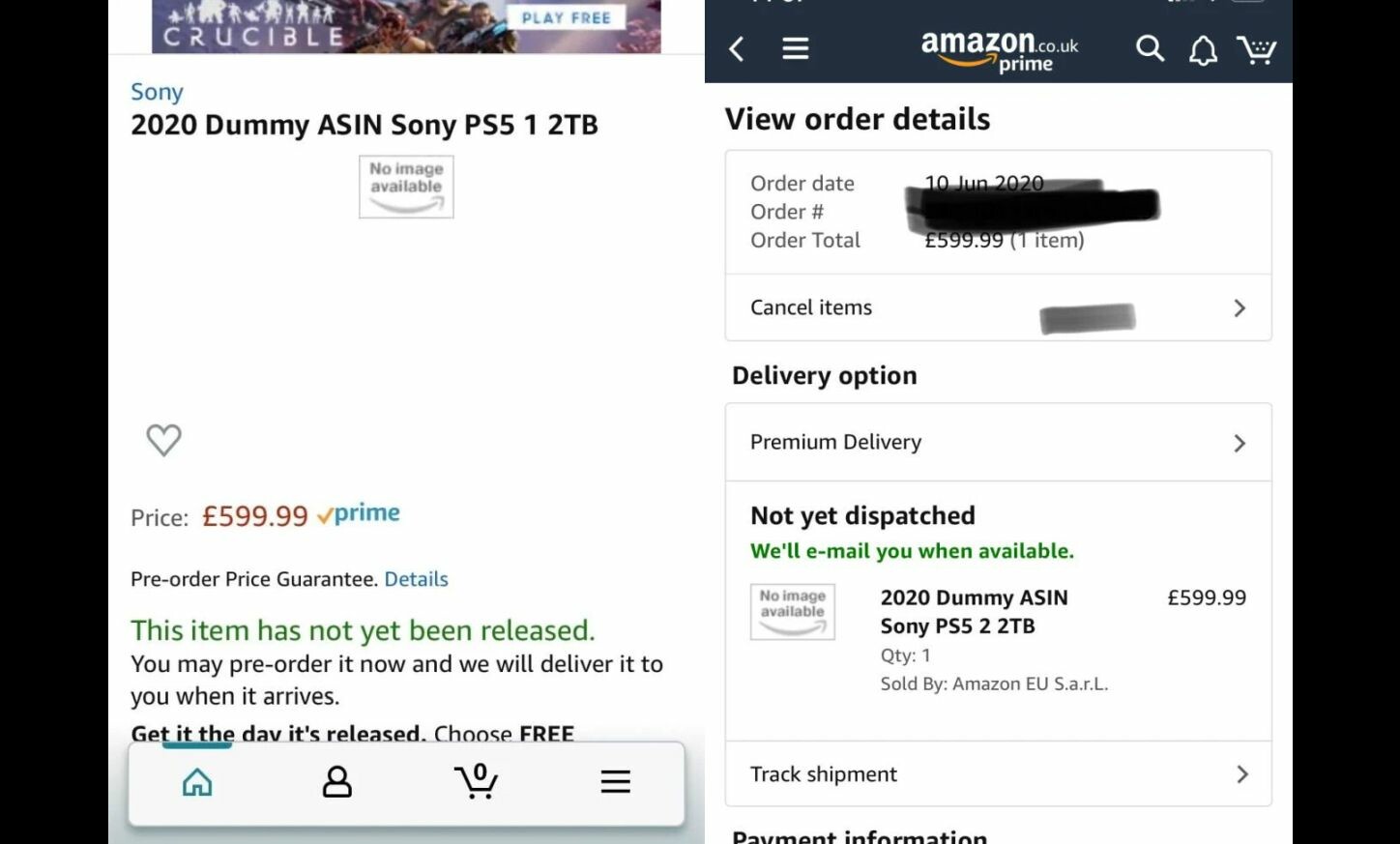**Detailed Descriptive Caption:**

On a solid black background, there are two distinct screenshots side by side.

The first screenshot details a product listing for the Sony PS5. Key textual elements include:
- The title, "Crucible, PlayFree" highlighted in blue.
- The brand "Sony" also in blue.
- The description "2020 Dummy" followed by technical specifications such as "ASIN, Sony PS5, 1, 2TB".
- A placeholder square image with the text "No image available".
- Pricing information listed as "£599.99".
- A "Pre-order Price Guarantee" notification.
- Further details presented in blue and green text.
- A note in bold stating "This item has not yet been released. You may pre-order it now and we will deliver it to you when it arrives. Get it the day it's released."
- Options to "Choose" with the term "free" notably in bold.

The second screenshot captures a section of an order summary:
- Details like "Order Date: 10 June 2020".
- The order number obscured by a black scratch-out.
- The order total listed as "£599.99" for one item.
- A status update "Canceled items" with subsequent details grayed out.
- Delivery option mentioned as "Premium Delivery".
- A status in green text indicating "Not yet dispatched".
- A final message, "We'll email you when available."

This detailed imagery provides a glimpse into the pre-ordering and product listing experience for the highly anticipated Sony PS5.